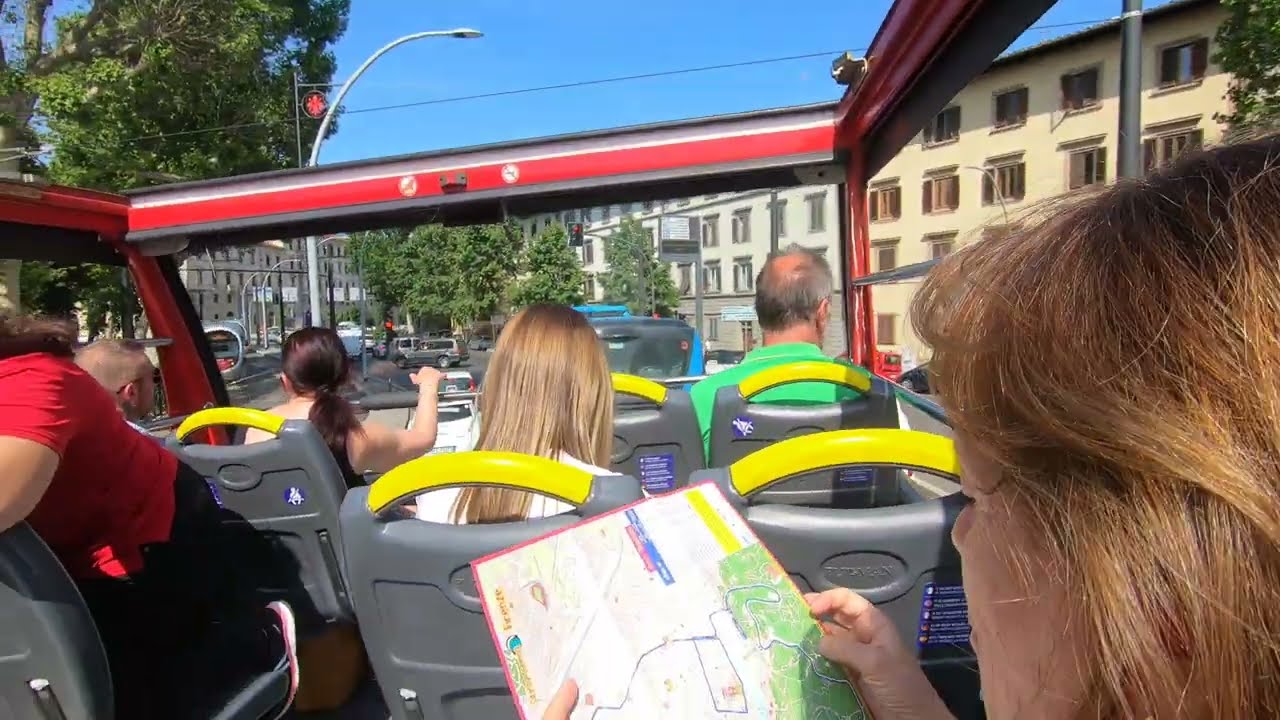This horizontal rectangular photograph captures a group of tourists on the upper level of an open-top double-decker bus, traveling along a street in what appears to be a historical or European-style area. The image is taken from within the bus, showing the backs of the passengers. Prominently, a woman with reddish-brown hair sits in the lower right corner, holding a map and seemingly checking the route. The bus is equipped with gray seats that have yellow tops, and there is a distinct lack of windows, offering an unobstructed 360-degree view. To the left, partially visible is a person in a red t-shirt and black pants, while in the front, there is a blonde woman and a balding man in a green shirt. The bus appears to be at a stoplight, with the red light visible amidst the blue sky and the taller buildings in the background. Additional details include trees scattered among the buildings and light poles along the street, with minimal traffic and possibly other tour buses ahead.